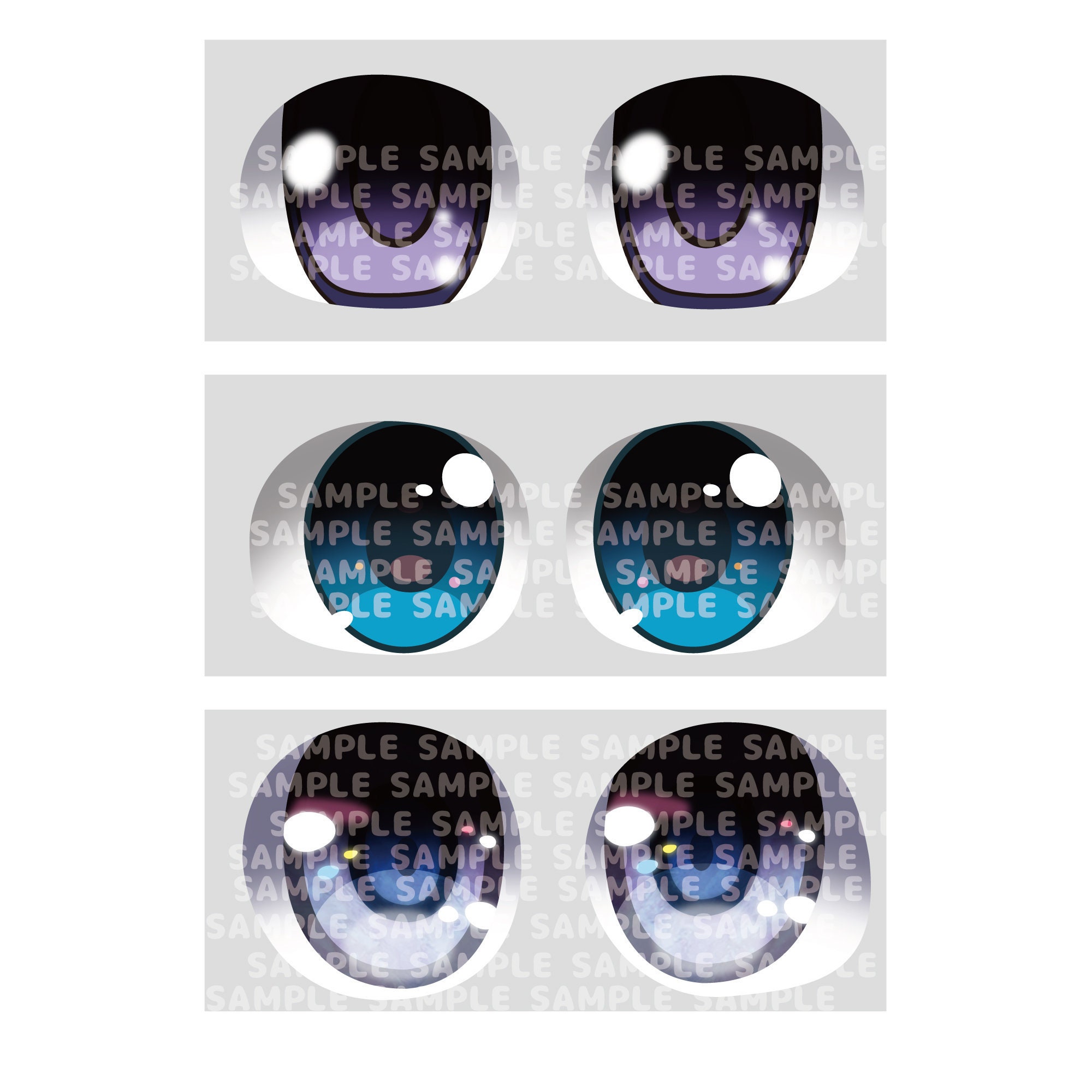The image consists of three computer-generated, cartoon-like sets of eyes stacked vertically, each with variations in color and specific light reflections. The background is a soft gray and each set is divided by white lines, giving the impression they're behind glass or encased in plastic. The word "SAMPLE" is repeatedly stamped across each set of eyes.

The top set features purple eyes with a distinct white spotlight effect in the top left corner of each eye. The middle set of eyes is turquoise-blue with a larger white reflection in the top right corner and smaller white circles throughout, creating a detailed light effect. The bottom set consists of primarily white eyes with hints of blue. They also feature multiple white circular light reflections, including notable spots in the top left and bottom right corners of the eyes. Each set has equal emphasis on the intricate light reflections and the overall softened, digital appearance.